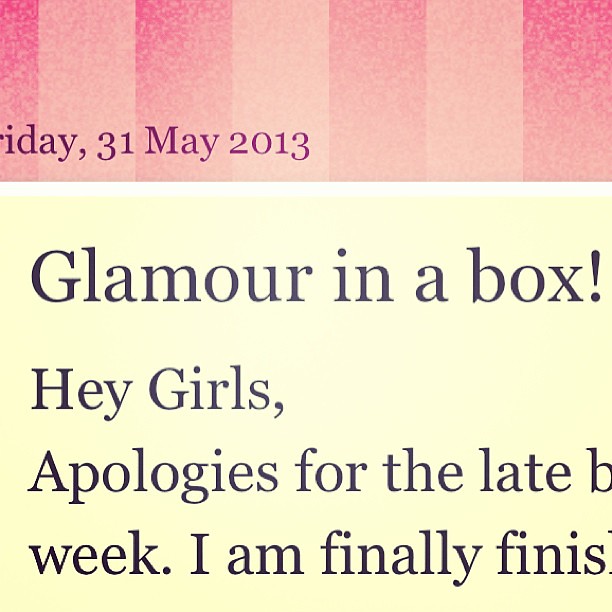The image depicts a close-up of a computer graphic, possibly an HTML email or a part of a web page. At the top third of the image, there is a banner with alternating vertical stripes in shades of reddish-yellow and yellowish-red. The banner features dark text that partially reads "Friday 31 May 2013," with the "FR" in "Friday" truncated. Below the banner, a light yellow background occupies the lower portion of the image, presenting several lines of black text. The prominently visible text includes "glamour in a box!" followed by "Hey girls," with the next line reading "apologies for the late" but trailing off with a partially visible 'B'. The concluding text line begins with "week," followed by "I am finally," and what seems to be the word "finished," although the 'H' is cut off from view. The text appears to be directed towards a group of girls, possibly as part of a message or announcement.